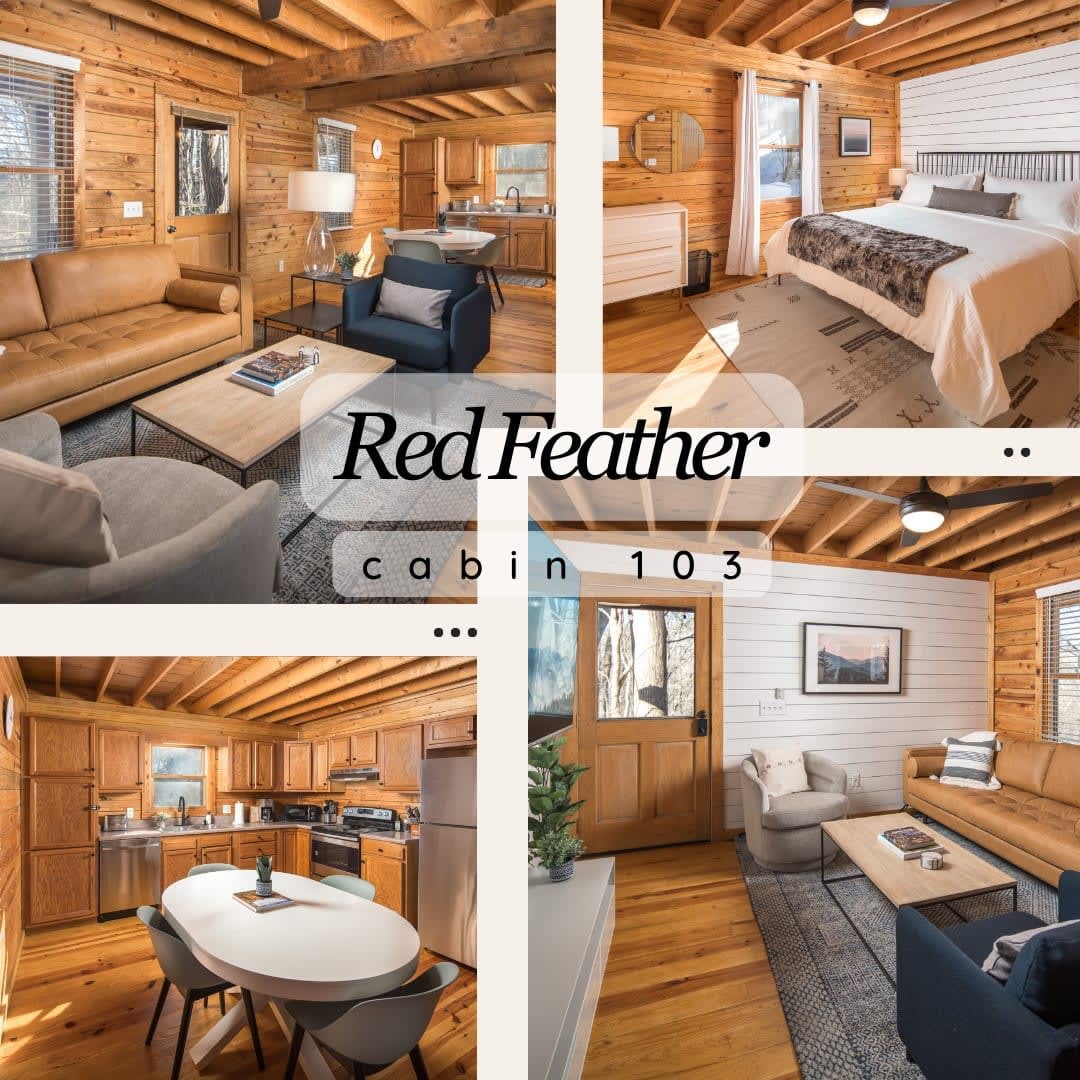The advertisement image for "Red Feather, Cabin 103" comprises four inviting photographs showcasing this charming tiny home. The upper left image highlights the cozy living room, featuring tan honey-colored wood paneling on the walls, ceiling, and floor. A large coffee table is surrounded by a cappuccino-brown leather couch, a gray chair, a small navy blue chair, and another chair, all accented by a gray area rug. The room is well-lit by a window in the upper left corner and a door with a window pane at the top.

To the upper right, there's a serene bedroom with white bedding, two plush pillows, and a blanket. Behind the bed, the wood-paneled wall is painted white, creating a peaceful contrast. The bedroom is further accessorized with a gray rug, a desk, and a mirror. A window with white curtains adds to the room's tranquility.

The lower left photo provides a close-up of the fully equipped kitchen. All cabinetry matches the same honey-colored wood theme, complemented by stainless steel appliances. An oval white table sits in the middle, surrounded by four chairs. 

Finally, the lower right image offers another perspective of the living room, this time including the back door. This angle reveals a section of the wall painted white, along with the door featuring a window for added natural light. 

These four images combined give a comprehensive and warm portrayal of the inviting "Red Feather, Cabin 103."